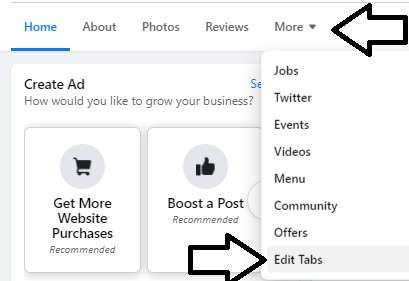The image depicts a screen capture from an online application page, specifically showcasing the navigation menu options. At the top of the page, the menu options are aligned horizontally. The "Home" option, prominently underlined in blue, occupies the top left corner. Directly to the right of "Home," in grey text, are additional menu items listed sequentially: "About," "Photos," "Reviews," and "More." 

The "More" option features a drop-down arrow indicating further selections. Below this main horizontal navigation bar, an additional vertical menu lists several options starting from the top: "Jobs," "Twitter," "Events," "Videos," "Menu," "Community," "Offers," "Edit," and "Tabs."

Dominating the left side of the image, directly below the highlighted "Home" option, is the main content area characterized by a white background. Within this section, bold black text reads "Create" and "Add." Beneath these headings, smaller grey text poses a question: "How would you like to grow your businesses?"